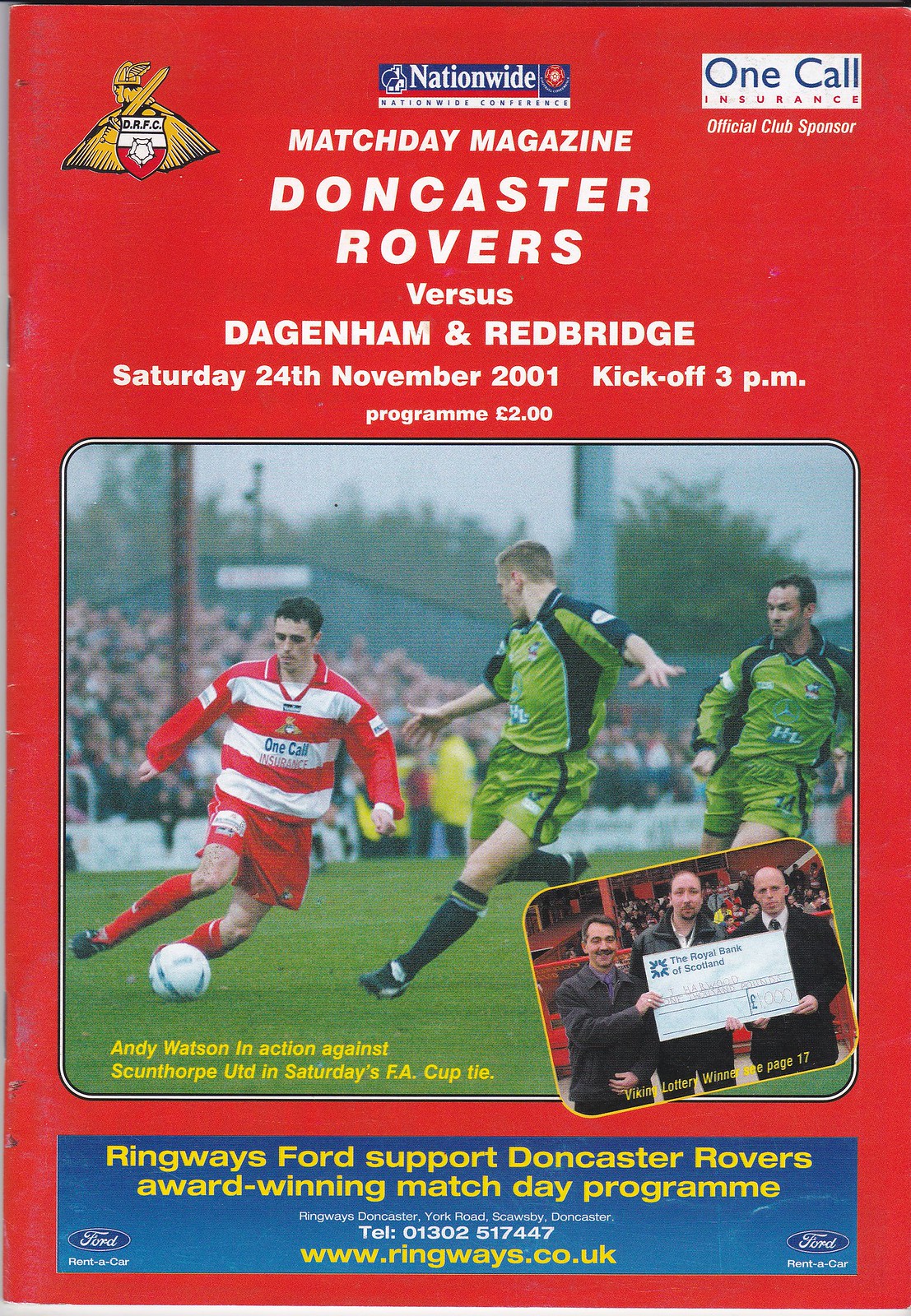The vibrant red poster serves as the cover for the Match Day Magazine featuring a football match between Doncaster Rovers and Dagenham & Redbridge scheduled for Saturday, 24th November 2001, with a 3 p.m. kickoff. Priced at two pounds, the program includes contact information and sponsorship details. Central to the design is an action photograph of three soccer players on the field. One player, clad in a red and white horizontally striped jersey, red shorts, and red socks, is seen kicking the ball. He is flanked by two opponents in green and black jerseys and shorts. This action shot is set against the backdrop of stadium stands filled with spectators. The top of the poster prominently features the match details in white typography, while the bottom includes a blue rectangle with yellow text promoting Ringways Ford and displaying a telephone number and website. Additionally, a smaller inset photo at the bottom right captures three men holding a white donation check. The overall style merges photographic realism with graphic design elements, creating a visually engaging program cover.